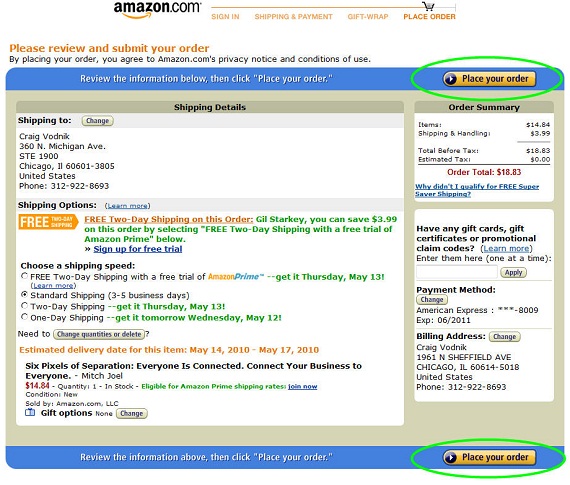The top section of the image features the text "amazon.com." Below, it reads, "Please review and submit your order. By placing your order, you agree to the amazon.com privacy notice and conditions of use." Further down, it instructs, "Review the information below and click 'Place your order.'" Below this, there's a prominent yellow button that has a black oval with a play icon inside and the text "Place your order." 

The yellow button is encircled by a hand-drawn green oval. Additionally, there is a similar visual marker around another button at the bottom of the image. Directly beneath the primary yellow button, the text "Shipping details" is visible. It specifies that the shipping is addressed to Craig Vognik at 260 North Michigan Avenue, Suite 900, Chicago, Illinois, 60601-3805, United States. The contact number provided is 312-922-8693. The image notes that the order qualifies for free shipping with free two-day shipping. It also suggests that Gil Starkey could save $3.99 on this order by selecting free two-day shipping with a free trial of Amazon Prime.